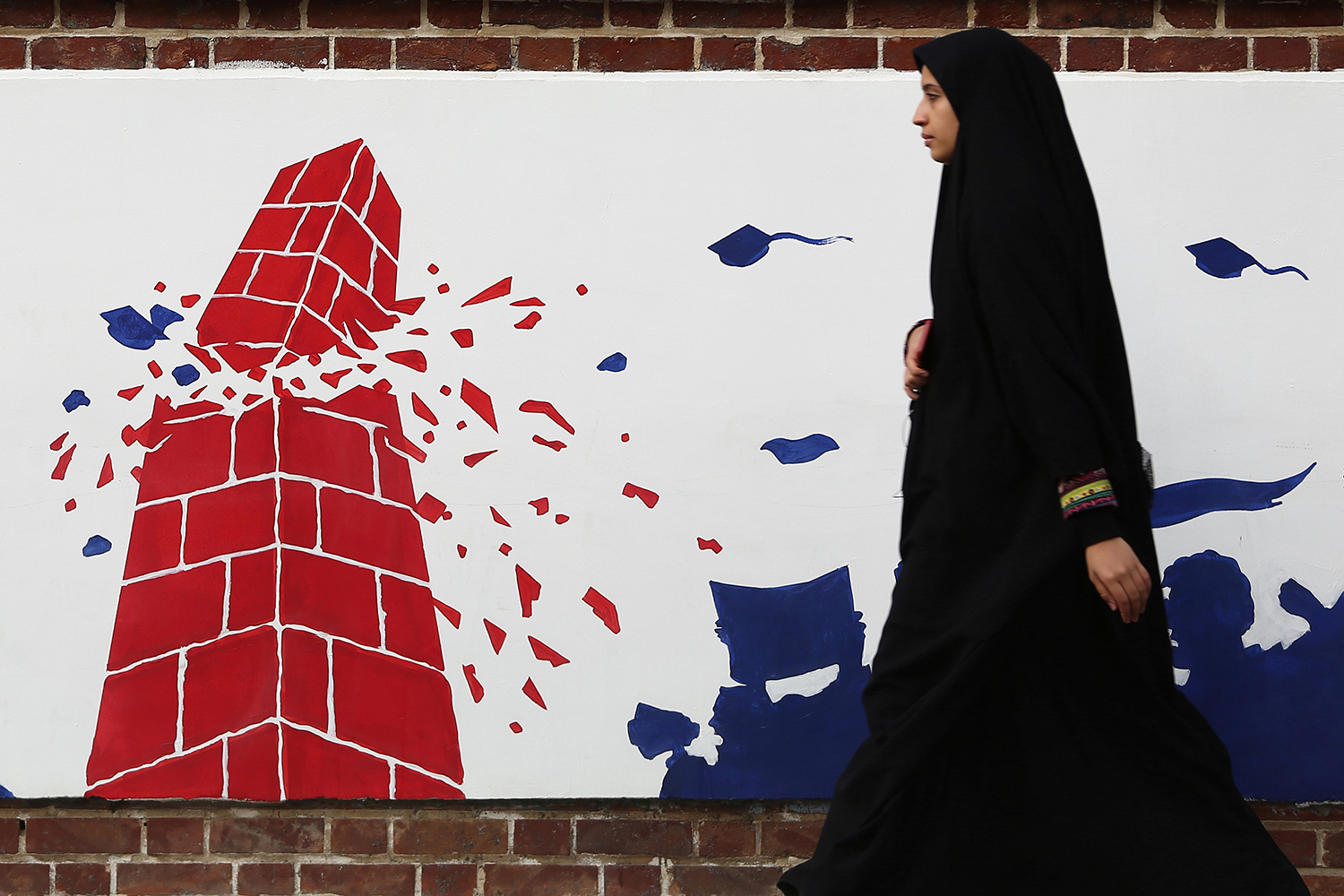This image showcases a detailed portrayal of a painting mounted on a brick wall, identifiable by the visible mortar lines between the bricks. The painting itself features a white background with a depiction of a partially collapsed four-corner brick wall on the left side, visibly cracked in the center with diamond-shaped fragments cascading down. To the right of this crumbling structure, an angry mob of people is depicted, hurling objects that appear to contribute to the wall's destruction. Outside of the painting, a person dressed in traditional Muslim attire, including a hijab covering their hair and a long black dress, is shown walking past the artwork. The combination of the painting's vivid imagery and the observer adds depth and context to the scene.